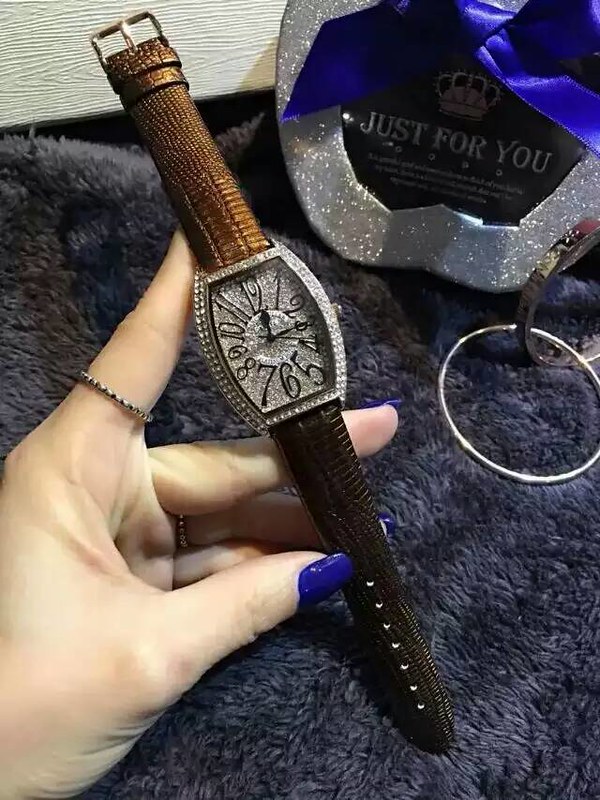The photograph, taken indoors, features a visually striking composition set against a backdrop of dark blue, fur-textured cloth. At the center of the scene is a luxurious gift box adorned with a blue bow intricately edged in sparkling silver. The box itself is black with elegant silver lettering that reads "Just for you." Adding a regal touch, a silver crown is perched atop the box. Complementing the opulent display are two metal hoops, interlinked and shimmering in silver, placed beside the box.

On the left side of the image, a woman's hand is partially visible. Her fingers, adorned with silver rings and painted with blue nail polish, gently grasp a watch. The watch is distinguished by its brown leather wrist strap and dazzling gem-encrusted face. Black numerals are clearly visible on the watch face, with matching black hour, minute, and second hands completing the timepiece's sophisticated design.